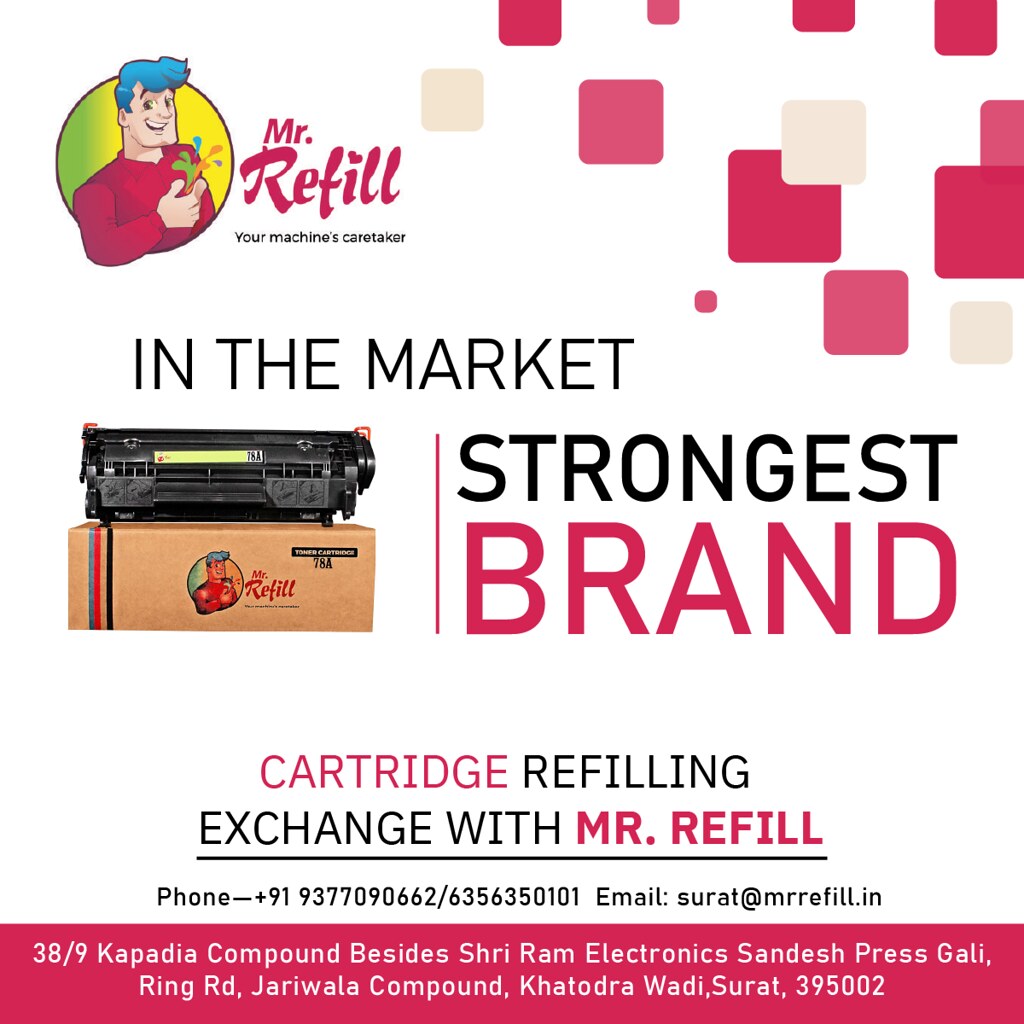This advertisement features Mr. Refill, presented on a predominantly white background. In the top left corner, a black-outlined circle contains a cartoon image of a muscular man with blue wavy hair, wearing a red shirt. The man is depicted holding colorful, liquid-like magic emanating from his hand. Next to the circle, the words "Mr. Refill" are prominently displayed in red letters, followed by the phrase "your machine's caretaker" in smaller black print. A design of pink and red squares lies to the right of this text. Below, black lettering reads "in the market." Further down is an image of an electronic device resembling a printer toner, placed on a box bearing the Mr. Refill insignia and name. A vertical pink line divides the advertisement, leading to the phrase "strongest brand" in black and large red letters respectively. The ad continues with the lines "cartridge refilling" and "exchange with Mr. Refill," followed by a black horizontal line and contact information, including a phone number, email address, and a red rectangle stretching across the bottom of the ad with additional white text likely listing an address.